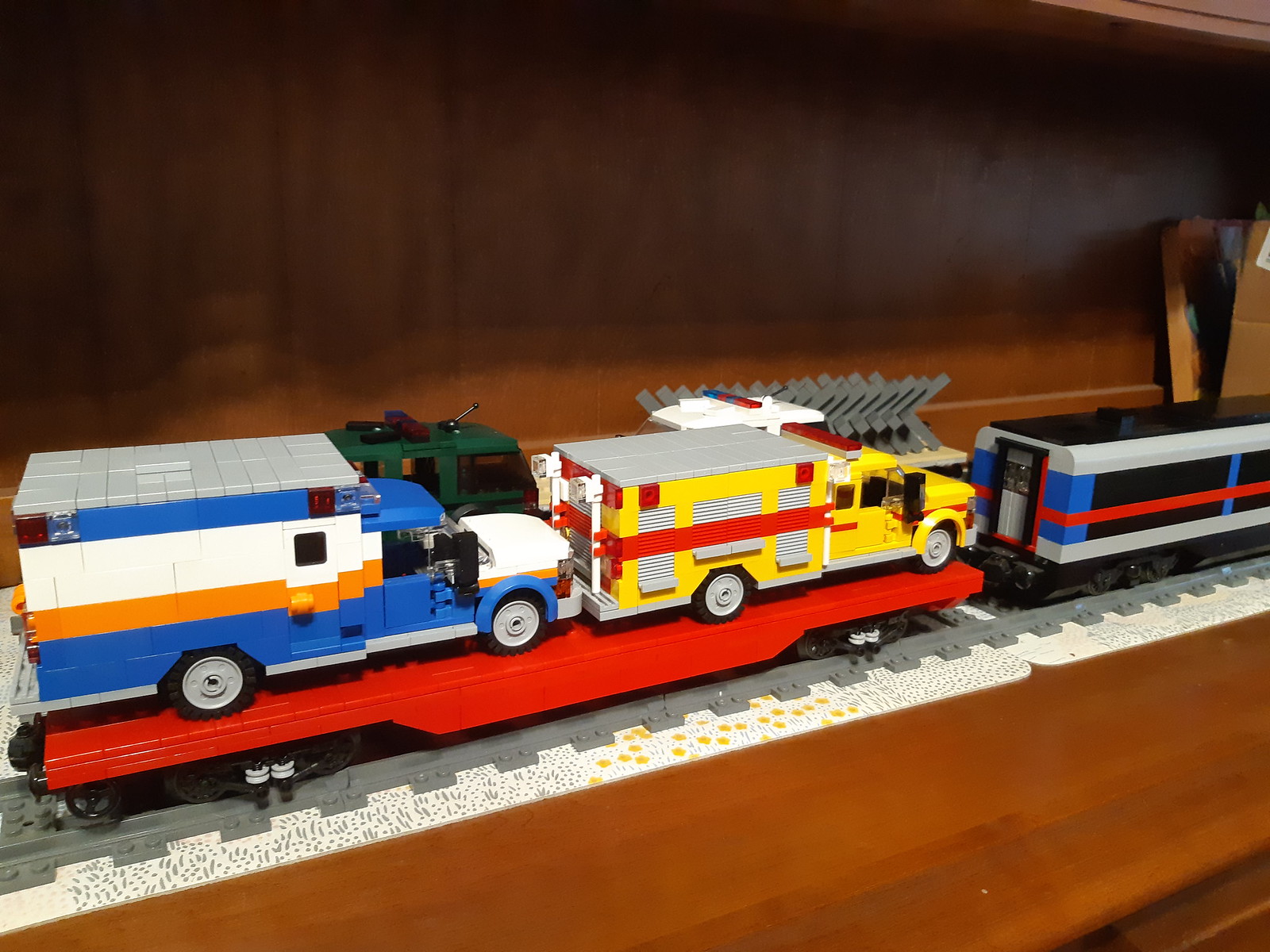This color photograph, taken in landscape orientation on a wooden table with a wooden backdrop, showcases a detailed scene of Lego vehicles arranged on plastic train tracks. At the forefront of the image is a gray, black, blue, and red Lego train car. Directly behind it is a red flatbed rail car, also made of Lego, carrying two Lego trucks: a yellow truck with a red stripe, and a white truck with orange and blue stripes, resembling ambulances. All the vehicles are intricately assembled from interlocking bricks, likely Lego or a similar brand. The entire setup is meticulously placed on gray toy train tracks, emphasizing the playful yet precise arrangement of these model vehicles.